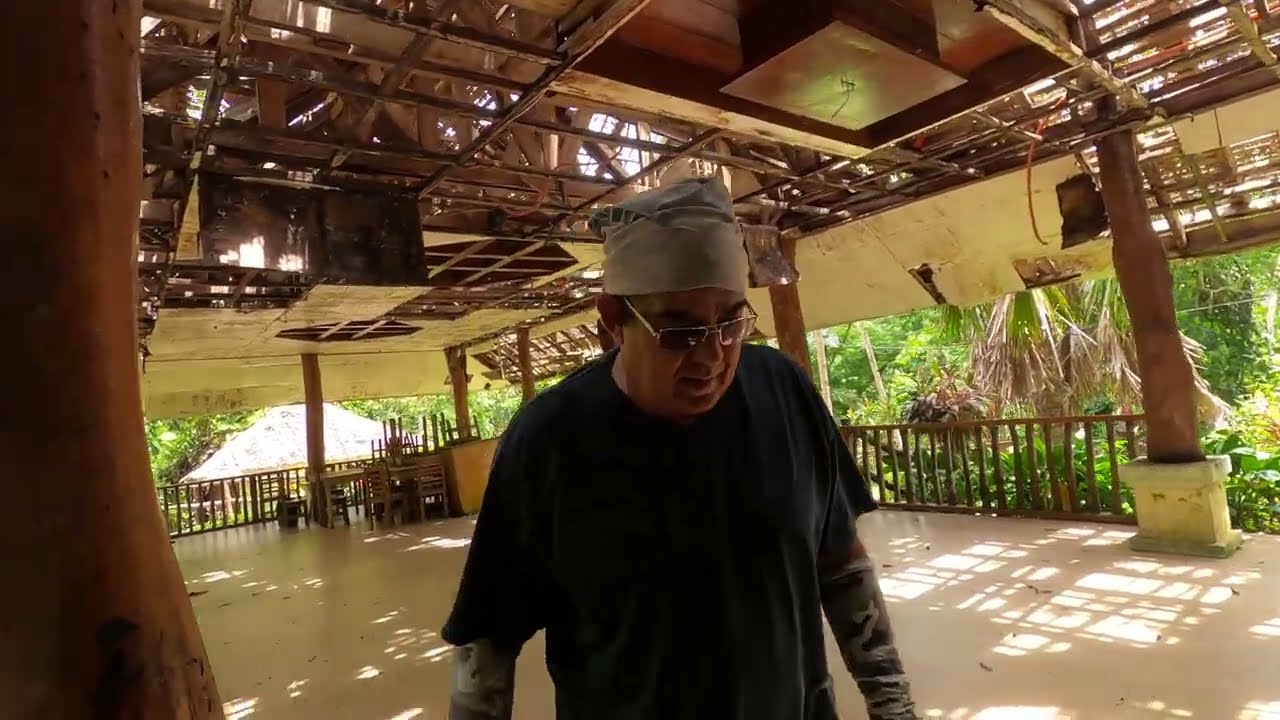In this image, an older white man, likely in his late 50s, stands beneath a large outdoor pavilion. The structure has no walls and is supported by numerous wooden pillars, creating a spacious and open environment that could easily accommodate dozens of people. The roof of the pavilion is complex, featuring a network of girders, rails, and various horizontal and vertical beams.

The man is dressed in a black t-shirt and wears a cloth or do-rag on his head, which could be mistaken for a chef's cap. He also sports glasses or sunglasses and appears to have either tattoos on his arms or is wearing camo-colored sleeves. Both of his hands are covered with some kind of cloth. 

Directly behind him, a wooden fence marks the boundary of the floor, beyond which lies a vibrant and dense jungle with palm trees that suggest a tropical setting. The sunlight filtering through the overhead grid-work of the roof casts sharp, downward-angled shadows, indicating it is the middle of the day. In the background, there is also a structure resembling a wooden hut with an angled roof, adding to the impression of a scenic, possibly tourist-oriented locale.